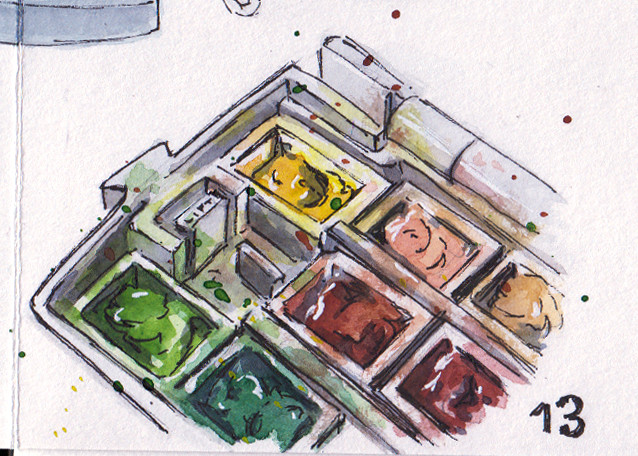The image is a detailed painting on a thick, rough-textured white paper marked with the number 13 at the bottom right corner. The painting depicts a compartmentalized tray, resembling an ice cube holder or a box for holding items, with parts of the tray slightly faded towards the edges of the page. The tray contains seven vats filled with colorful substances, each appearing almost like gelatin or liquid. The vats are filled with a light green, a darker green, two shades of red, yellow, a pink (skin type), and a brownish yellow. There are splotches of these colors across the tray and scattered on the white background around it, adding to the overall vibrancy of the image. Additionally, the word "lift" is inscribed, hinting that it could be part of a larger illustration, possibly depicting an elevator shaft or a liftable door mechanism. The painting's detailed depiction of shades and hues, along with the bleed of colors beyond their respective containers, suggests a close-up section of a more extensive artwork still partially out of view.